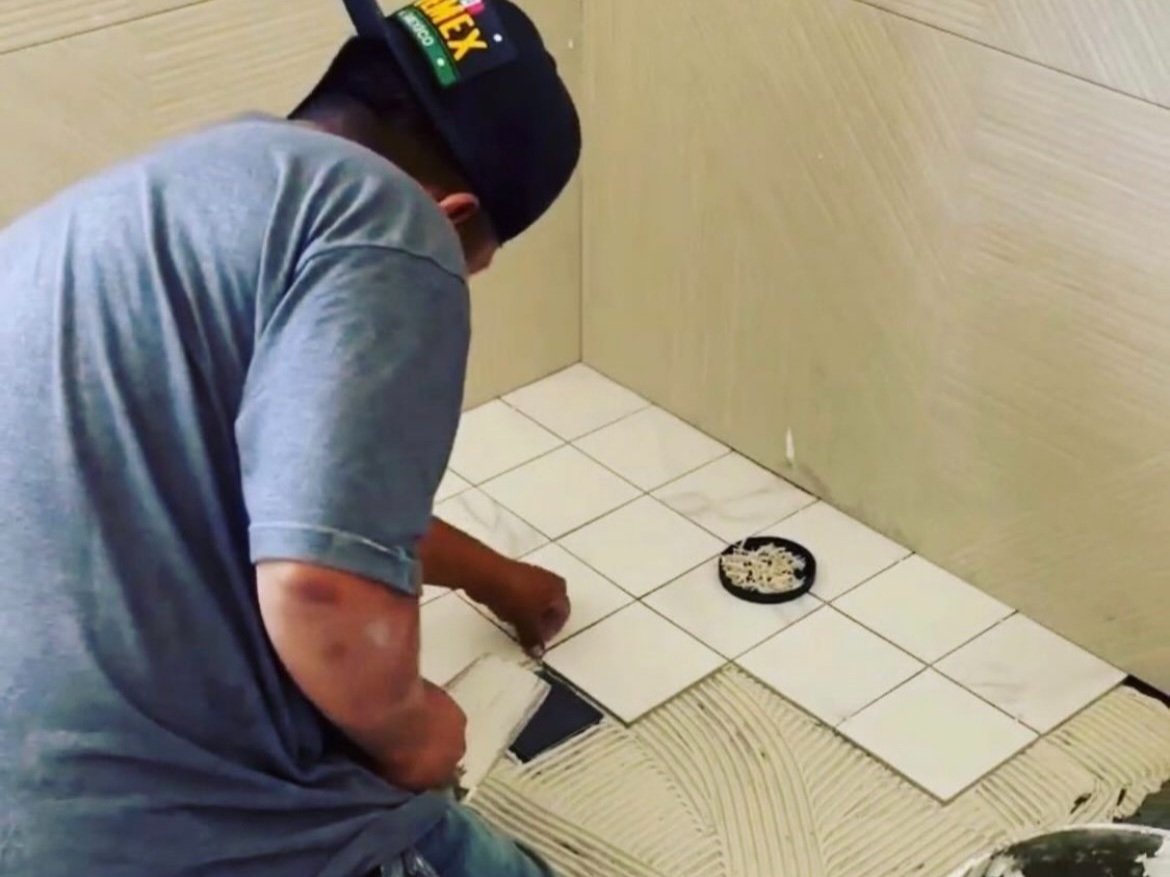The photograph captures an indoor scene where a man is seen engaging in some tiling work. Positioned on the left side of the image, the man is wearing a blue short-sleeved shirt and blue jeans, with a medium complexion. He sports a black hat turned backward, adorned with yellow text and a green box containing illegible text. The backdrop of the scene on the right side is a wooden wall with a warm, golden tone. 

On the floor, the man is meticulously placing white square tiles. Currently, there are two complete rows of six tiles each aligned against the wall. Adjacent to these, a third row is partially completed with four tiles already laid out. A black lid, likely from a container of tile adhesive, rests on top of the placed tiles. The lid has a notable amount of white adhesive stuck to it, indicating active use. The floor, covered in several tiles, showcases the man’s ongoing effort to renovate or complete the tiling project.